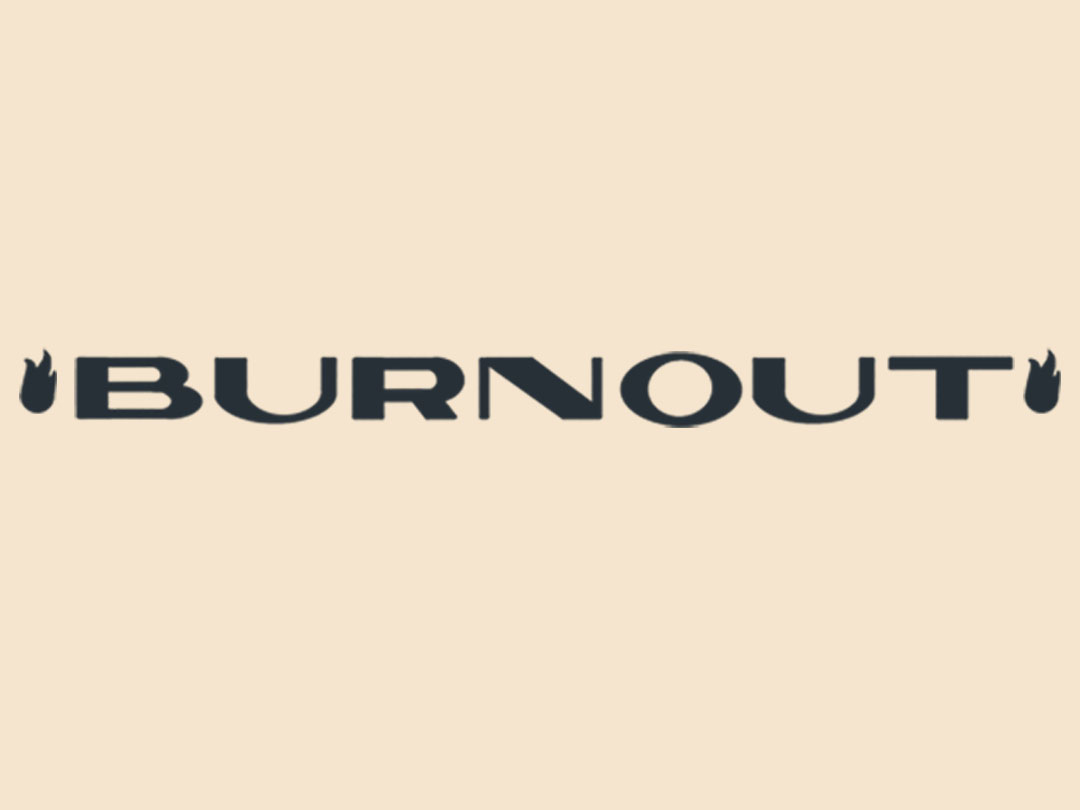This image is a graphic with a slightly landscaped rectangular shape, featuring a medium to light cream background. Dominating the center 10% of the image, spanning horizontally, is the word "BURNOUT" in bold, black, all-caps modern font. The typeface is designed with varying line thickness: for instance, the diagonal line in the 'N' is thick while the two vertical lines are thin, the right-hand side of the 'U' is thin and the left-hand side is thick, and the horizontal bar of the 'T' is thick in the middle but thin on the top. Flanking the word "BURNOUT" are two black flame graphics, resembling stylized candle flames, one positioned to the left of the "B" and the other to the right of the "T". The simplicity and minimalism of the design draw focus to the concept of burnout, accentuated visually by the stark black text and flame symbols against the subdued cream background.